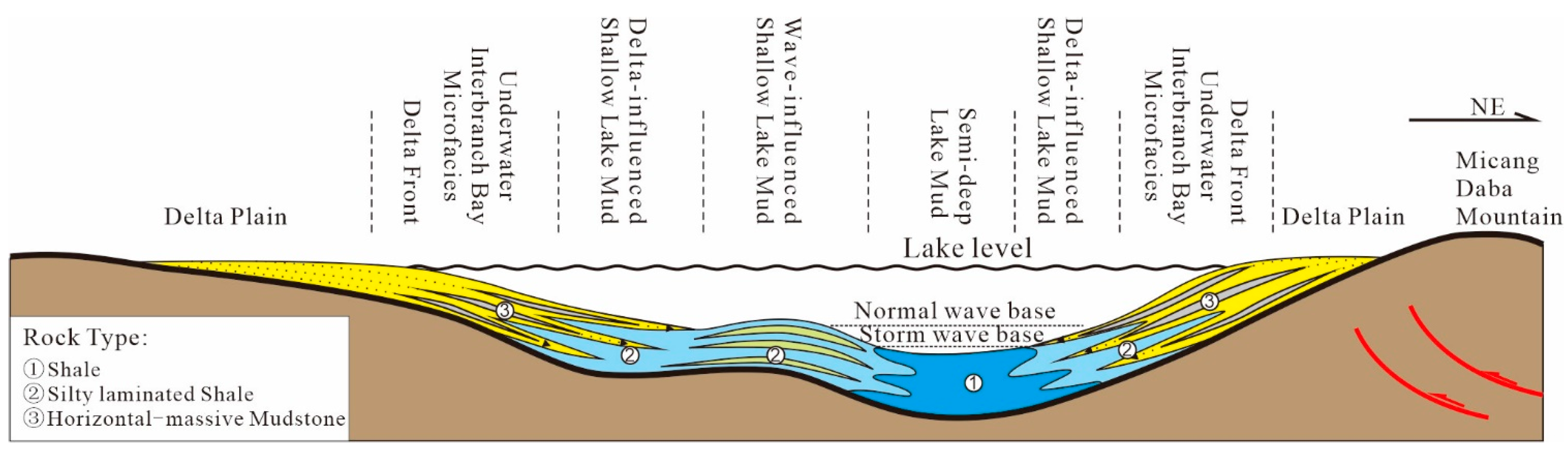This detailed infographic, likely from a textbook, illustrates the geological and sedimentary layers of a lake ecosystem. The horizontal print features a segmented landscape with varying rock types, specifically shale, silty laminated shale, and horizontal massive mudstone, as indicated in the lower left corner. The base layer is shaded brown, representing the Delta Plain, which slopes downward. The surface of this region is marked by yellow and blue lines signifying different water interactions.

Across the center of the image, a bold line indicates the lake level, above which water is depicted through various shades of blue. The lake's depiction includes sediments and formations such as the underwater interbranch bay, microfacies, delta front, delta influence shallow lake mud, wave influence shallow lake mud, and semi-deep lake mud. These labels, written vertically and sometimes sideways, categorize the different sedimentary environments within the lake.

To the right, the illustration extends to represent the Mekong Daba mountain, showing the transition from the Delta Plain to deeper lake regions. The infographic also differentiates between the normal wave base and the storm wave base through horizontal lines across the lake depiction, clarifying the impact of various wave activities on sediment dispersal.